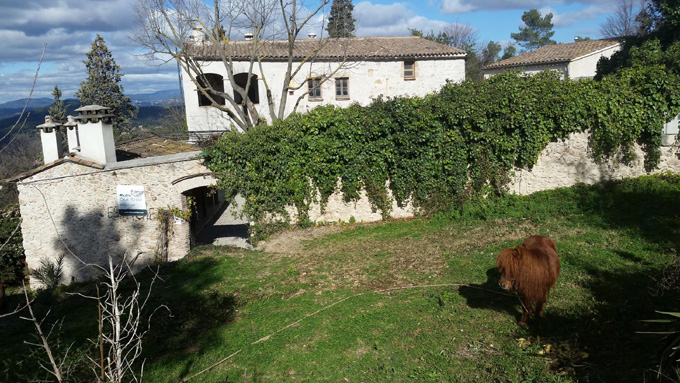In this daytime image, the scene captures a villa-style stuccoed house from a slightly elevated perspective, under a clear sky with puffy white clouds. The house, reminiscent of architecture seen in Spain or Italy, features a gray clay tile roof. To the left of the main villa, there's a smaller house with a high triangular roof adorned with three distinct chimneys or exhaust stacks. In the foreground stands a white stone entrance gate, partially covered in dark green ivy and overgrown shrubs. To the right, a shaggy brown Shetland pony, roped and tied, gazes to the left. The leafless trees just behind the gate add an additional layer of depth to the tranquil rural setting.